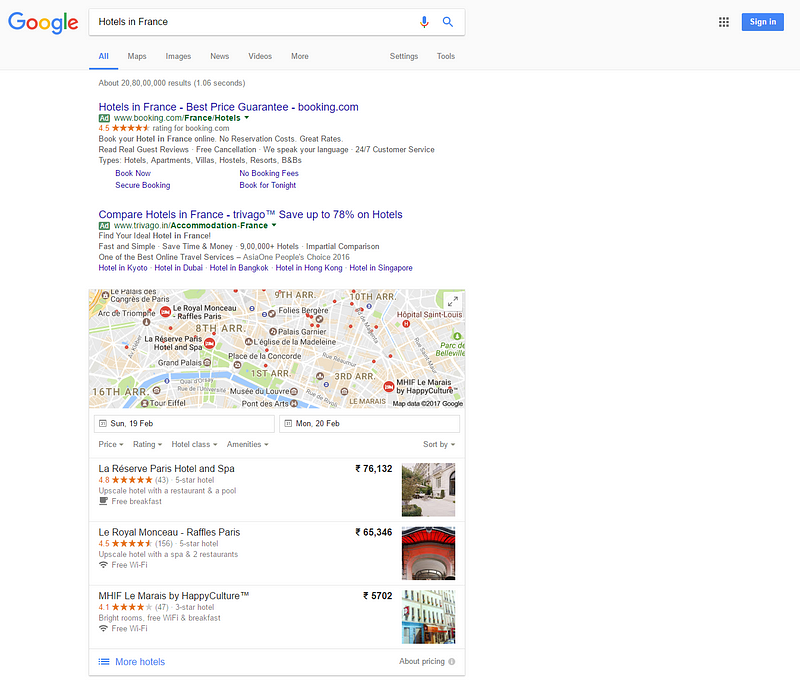"Google search results for 'hotels in France' are displayed in the 'All' tab, highlighting two advertisements. The first ad features Booking.com with a 'best price guarantee' label, while the second promotes Trivago, offering savings of up to 78% on hotel bookings. Below the ads, an area in France is showcased, pinpointing main attractions. Three hotel options are presented: 
1. La Réserve Paris Hotel and Spa, rated 4.6 stars based on 43 reviews.
2. La Royal Monceau - Raffles Paris, rated 4.5 stars from 156 reviews.
3. Hotel MHIF Les Marais by HappyCulture, holding a 4.1-star rating.
The locations of these hotels are marked on a map, assisting users in visualizing their proximity to significant landmarks."